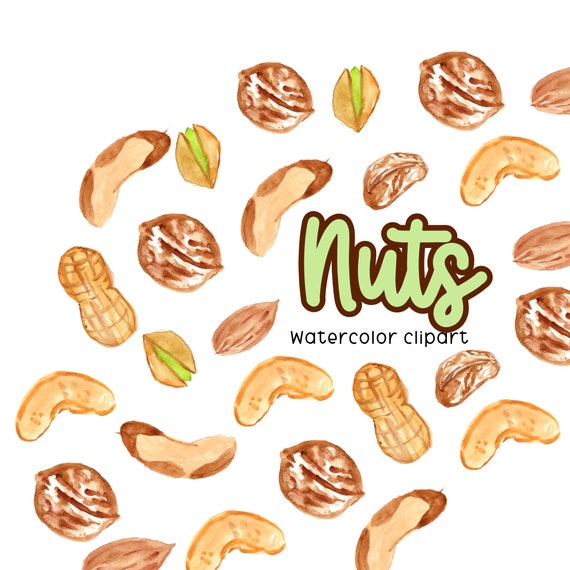The image showcases an array of various nuts illustrated in watercolor style, set against a pristine white background. Prominently in the center, the word "nuts" is elegantly scripted in pale green and outlined in brown. Below this, the text "Watercolor Clip Art" appears in black letters. Surrounding the central text, a diverse assortment of nuts, including walnuts, peanuts, cashews, almonds, pistachios with their distinct green centers, and possible pecans, are scattered. These nuts are depicted in various shades of light brown, tan, and darker brown, adding depth and texture to the composition. The overall effect is that of a detailed and artistic cover sheet for a collection of clip art, emphasizing the natural colors and distinct forms of each nut.